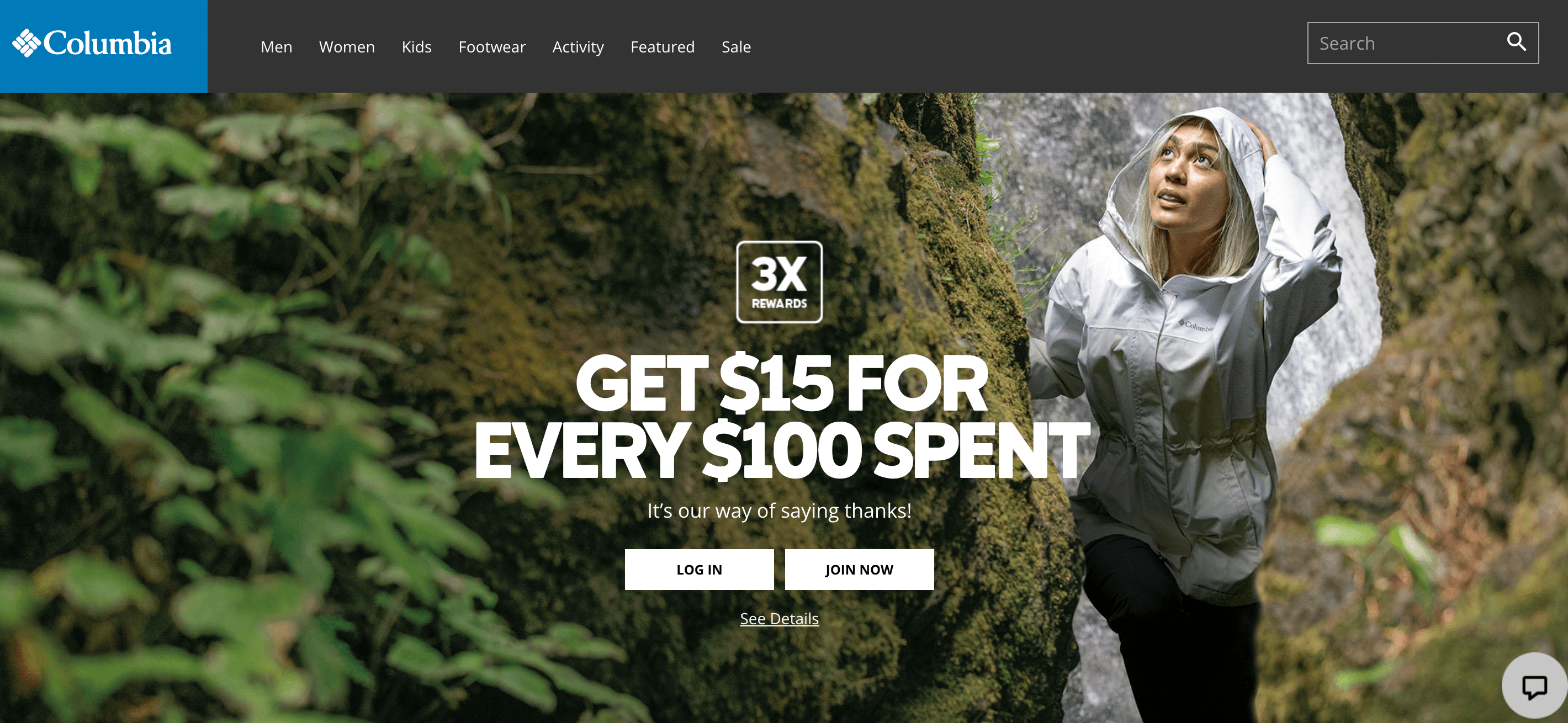The image features a webpage layout. At the top, a black navigation bar spans across the page. On the far left of the black bar, there's a small blue box displaying the word "Columbia" alongside the brand's logo. The navigation bar contains several menu buttons labeled in sequence: "Men's," "Women's," "Kids," "Footwear," "Activity," "Featured," and "Sale." Towards the far right end of the bar, there's a search box.

Below the navigation bar, the main image features a woman standing outdoors in a wooded area. She is wearing a parka with the hood up. The background includes a variety of natural elements: trees to the left and behind her, a mossy rock next to her on the left side, and another rock, either white or gray, positioned slightly behind her on the right.

Centrally positioned over the image is a promotional text in white, prominently displaying "3x 3x" with smaller, unreadable text beneath it. Further down, it reads, "Get $15 off for every $100 spent," followed by, "It's our way of saying thanks." Below this promotional message are two buttons labeled "Login" and "Join Now," with a "See Details" link underneath.